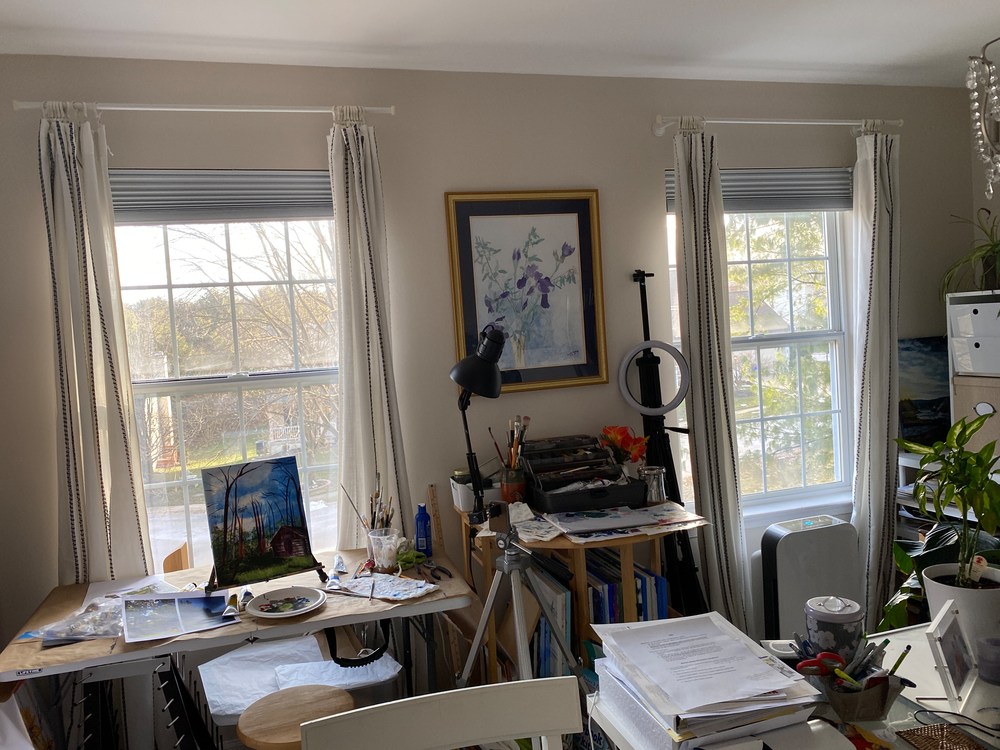The image depicts a cluttered home office filled with various objects and details. Dominating the scene are two desks, both untidy and brimming with items. The first desk, located towards the left, features a painting and sits beneath one of the two tall windows. Through this window, sunlight streams in, illuminating the entire room and revealing a view of trees outside. Adjacent to this desk, there's a basic wooden chair, and a stool nearby provides another seating option. The second desk, sitting in the center, is also cluttered with paintbrushes, books, a lamp, and numerous papers. Beneath this desk, there's a mini-shelf, adding to the general disarray. A potted plant rests in the corner by this desk, and two manila binders, one black and one white, are visible on the floor beside it. On the wall painted grey, above the second desk, a painting of various flowers hangs. Additionally, an air conditioner unit is mounted on one of the white walls, and an air purifier is positioned nearby. The room also features tall windows with curtains pulled all the way open, further enhancing the light and giving the space an airy, if disorderly, feel. Finally, a bright blue bottle, indicative of clutter, is somewhere in the mix, contributing to the overall impression of a busy, yet lived-in, home office space.